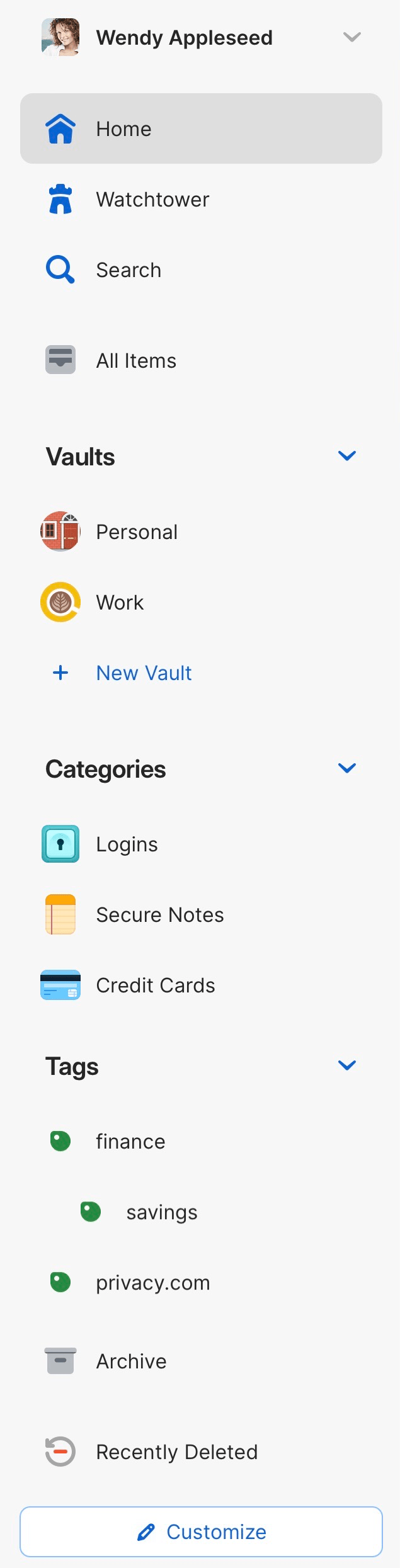The image depicts a detailed screenshot of a left-hand sidebar from a website with a minimalistic, light grey background. At the top, there is a small avatar icon of a woman's face labeled "Wendy Appleseed Bowl," accompanied by a drop-down menu. 

Below this, the navigation is sectioned into various categories, each with distinct icons on the left side. The initial section includes four sequential options: "Home," "Watchtower," "Search," and "All Items."

Afterward, there is a category titled "Vaults," which features a drop-down menu revealing sub-options: "Personal," "Work," and "New Vault." The "New Vault" option has a plus sign icon to indicate the possibility of adding a new vault.

The next category is "Categories," which also has a drop-down menu. Under this, options like "Login," "Secure Notes," and "Credit Card" are listed, each with corresponding icons.

Further down, there is a "Tags" section encompassing subcategories such as "Finance" and "Savings," with the "Savings" label slightly indented to the right compared to "Finance." Below "Savings," "Privacy.com" is aligned with "Finance," and each item in this grouping is marked with a small round green icon.

Towards the bottom, "Archive" is listed under the tags section, marked with an archive icon. The last option in the list is "Recently Deleted," accompanied by a small icon.

At the very bottom of the sidebar, there is a white button labeled "Customize," featuring a small pencil icon on its left side, suggesting user customization features.